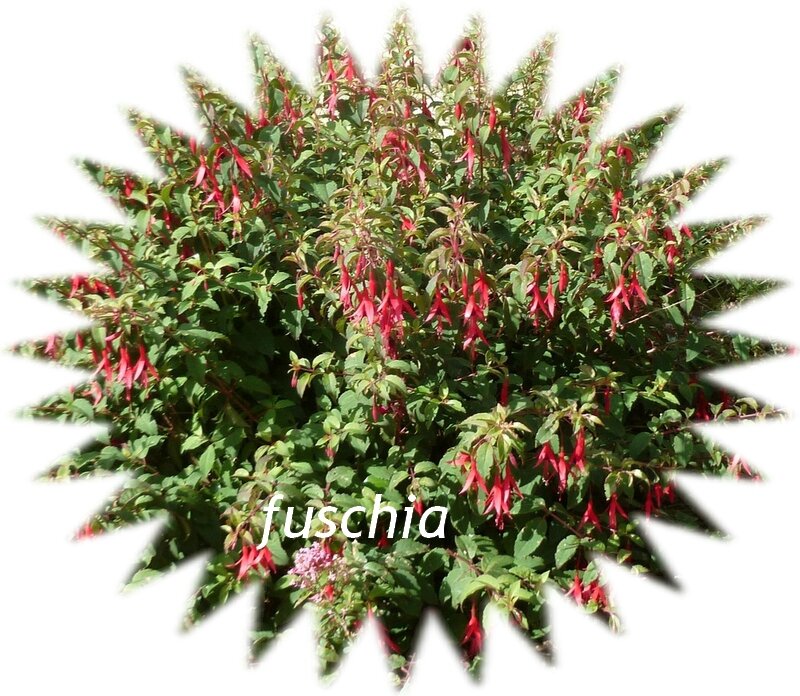The image depicts a vibrant fuchsia bush, prominently featuring lush green leaves and striking red flowers. The flowers, potentially of the fuchsia plant, hang elegantly with their long, thin petals cascading downwards and central pollen protruding delicately. The plant is visually centered against a green backdrop, creating a stark, lively contrast with the red blooms. Encircling the image is a unique starburst pattern with pointed edges, forming a sun-like white border that frames the photograph perfectly. The word "Fuchsia" is clearly overlaid in white text atop the center of the bush, suggesting either a botanical identification or an illustrative advertisement, possibly for seeds or gardening products.